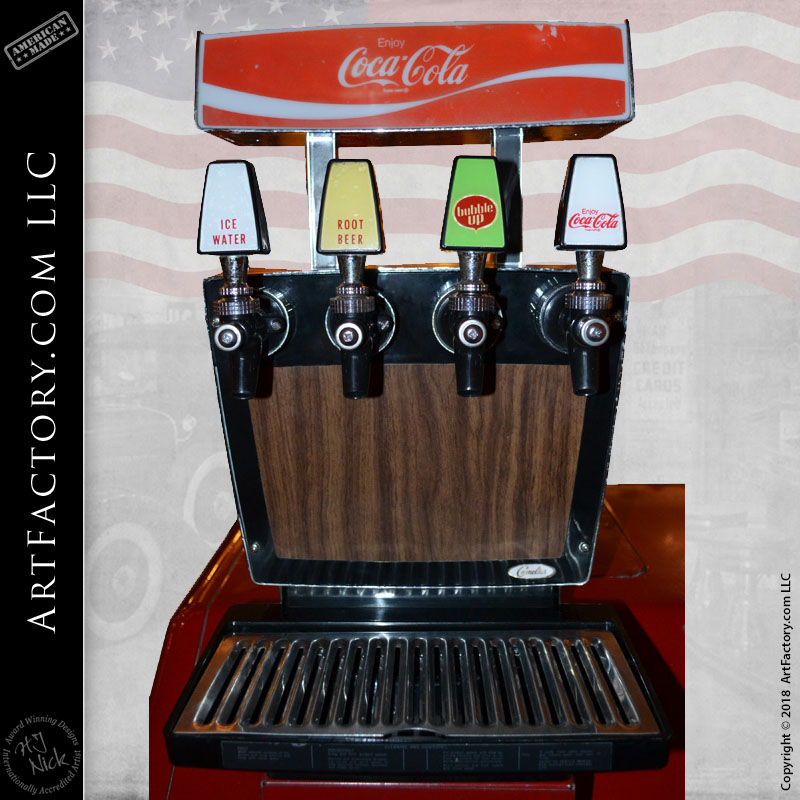This image features a classic soda dispenser set against a blurred background showcasing an American flag and an old-style car. The dispenser itself has a wood-paneled appearance and is predominantly black with four distinct spouts. The first spout is labeled for ice water, the second for root beer, the third for Bubble Up, and the fourth for Coca-Cola. Above these spouts, the iconic red and white Coca-Cola sign is prominently displayed, complete with the "Enjoy Coca-Cola" slogan and trademark symbol. The machine features a metal grate at the bottom for catching drips. On the left side of the image, the text "artifactory.com LLC" is written vertically and is followed by "American Made." Additionally, the machine carries a copyright designation from 2018 by Art Factory LLC.